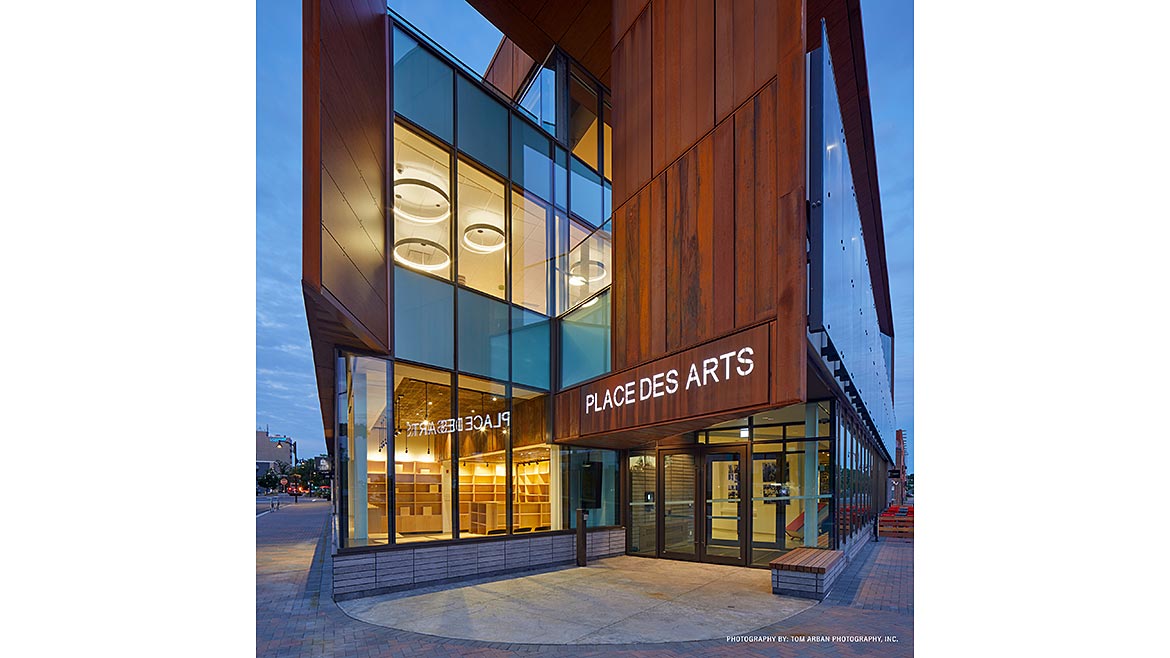The image depicts the entrance of the asymmetrical and predominantly glass building known as "Place des Arts." The building features a mix of brown wood paneling and large glass panes, creating a striking contrast. Above the entrance, the name "Place des Arts" is clearly displayed in white text. The entrance itself is primarily made of glass, contributing to the modern and transparent aesthetic of the structure. The building appears empty inside, illuminated by yellow lights. On the left side of the image, there's a view of the street with a lamppost and a car with its rear lights on. The scene is set in the evening, under a sliver of blue sky. Additionally, the left-hand side windows reflect parts of the street and surrounding architecture. The ground floor windows are fully transparent, while the second-floor windows have a design with alternating blue and clear sections. At the bottom right of the image, the credit "Photography by Tom Arban Photography, INC." is visible.